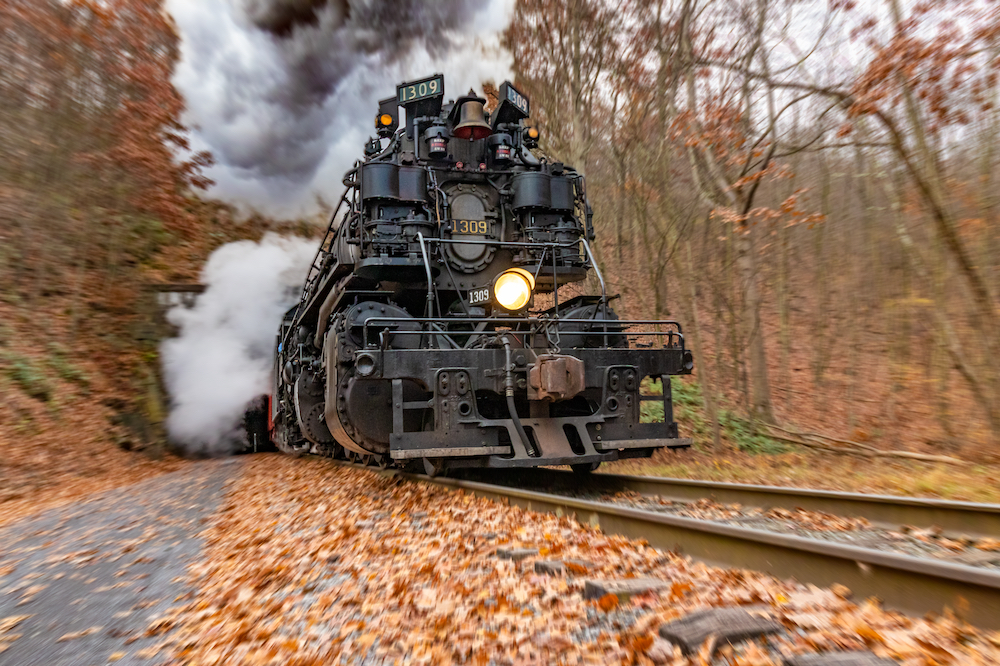The image captures a locomotive train engine with the number 1309 prominently displayed on the front. The train, painted black with some rusty areas, is moving through a wooded area on a fall day. The central headlight is illuminated with a bright yellow glow, cutting through the scene. The engine is releasing abundant smoke from its top and back, obscuring the background. Beneath the train, parts of the railroad track's wooden pillars are visible, though they are partially covered by fallen leaves. The surrounding trees are barren, with a mix of dead leaves on the ground and sparse patches of green. The motion of the train is evident as it is in focus while the surrounding wooded scenery appears blurred. There also seems to be a bell on the top front of the locomotive, adding to the detailed historical look of the scene. The sky overhead appears cloudy and gray, enhancing the autumnal atmosphere.